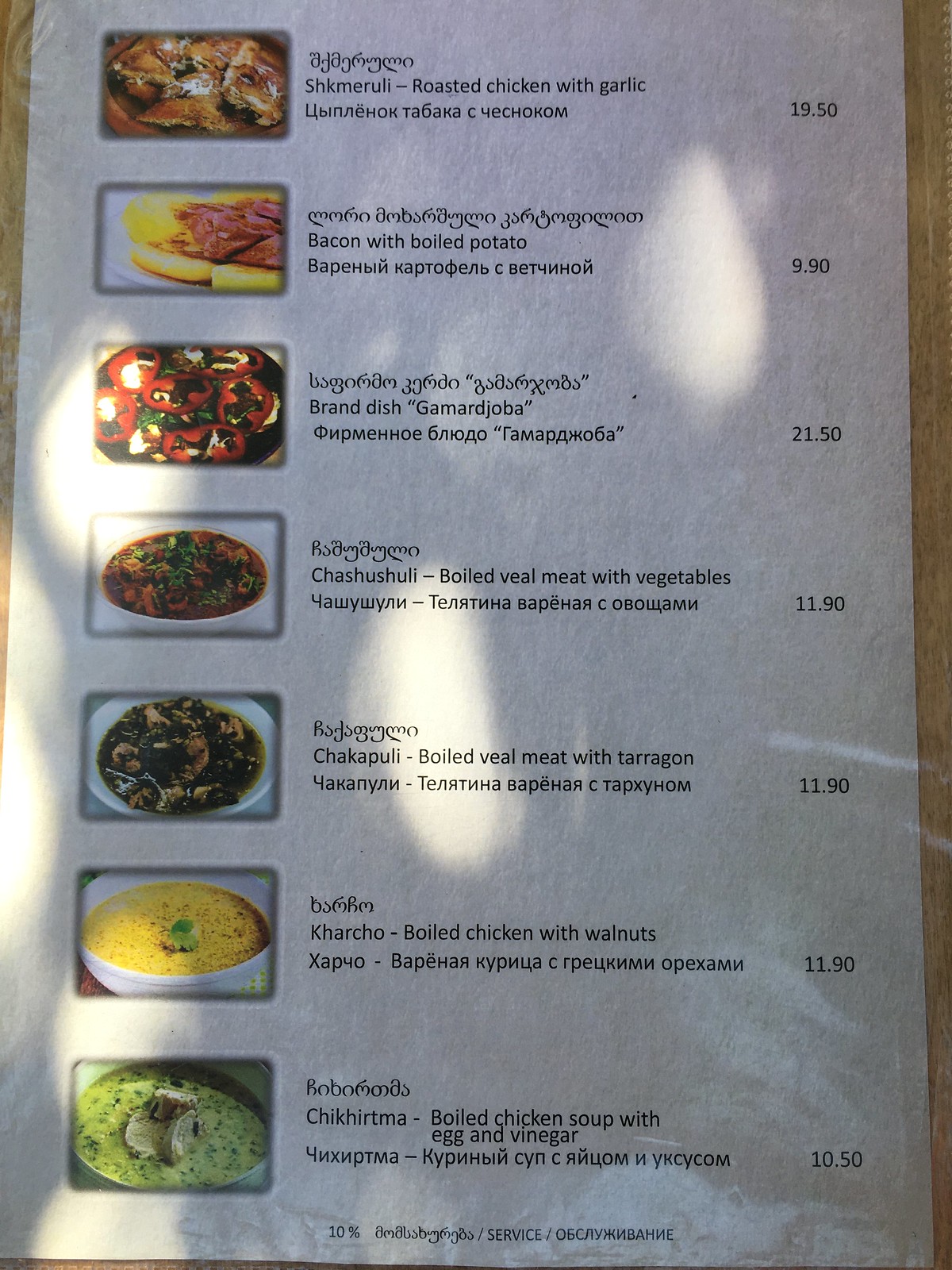This vertical color photograph captures a single white paper menu, subtly illuminated by scattered sunlight. The unlaminated page, absorbing the light, showcases seven menu items, each represented by a color photograph aligned in the left column. Adjacent to each image is a description in English and another language, accompanied by a price listed on the right. 

The menu begins with "Roasted Chicken with Garlic," followed by "Bacon with Boiled Potato." Further down are "Brand Dish Gamanjoba," "Boiled Veal Meat with Vegetables," "Boiled Veal Meat with Tarragon," "Boiled Chicken with Walnuts," and "Boiled Chicken Soup with Egg and Vinegar." Prices for these dishes range from $10.50 to $19.50. Each photograph is framed by a gray rectangular border, enhancing their presentation beneath the delicate sunlight dapples.